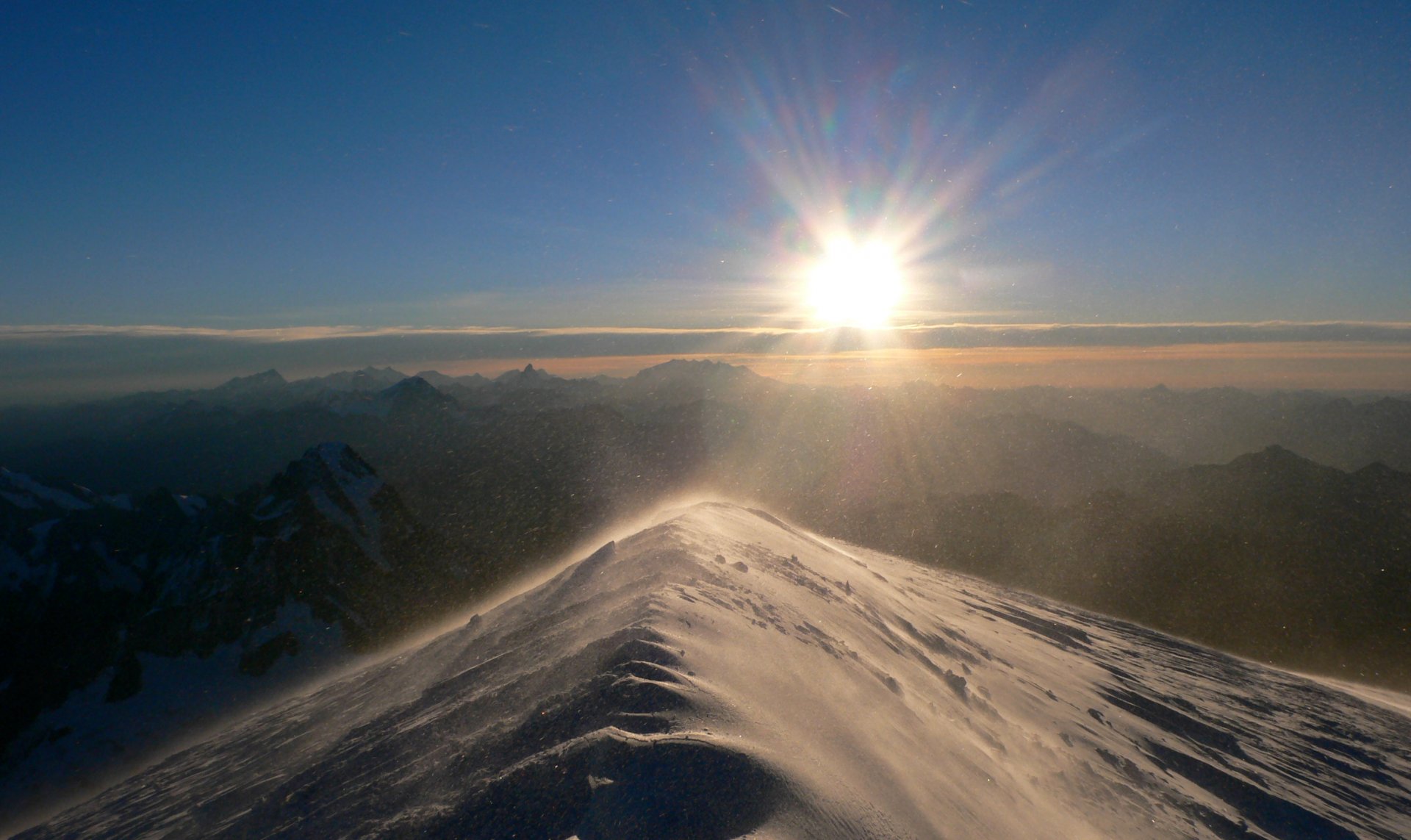This is a stunning, color photograph of a wintry mountaintop during sunset. The snow-covered peak occupies the foreground, with its slopes descending gracefully on both sides. The powerful gusts of wind lift a fine dusting of snow. To the left of this peak stands a slightly lower, snow-clad and dark stone peak, while to the right, an almost silhouetted peak frames the scene. The expansive mountain ranges in the background stretch as far as the eye can see, gradually becoming shadowed silhouettes that rise taller to the left of the sun, revealing hints of snow. The sun itself is brilliantly centered on the horizon, casting a blue tint over the entire landscape. Above, the clear sky transitions from light blue, through a band of white and blue clouds, to a burst of orange at the horizon. The serene yet cold environment perfectly captures the beauty of a wintry sunset over rugged mountain terrain.